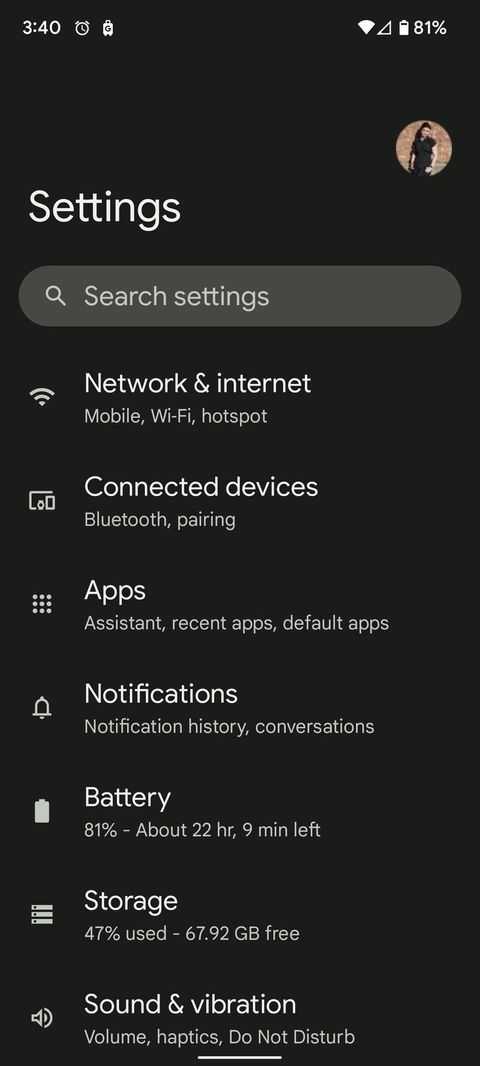The image depicts a smartphone's settings panel. The upper left corner showcases the time, reading 3:40, accompanied by an alarm clock icon and a lock icon. The full Wi-Fi signal is displayed, although the cellular reception is almost nonexistent, showing just about 80%. Adjacent to these details is a battery meter indicating 81% charge. A profile picture is visible, featuring a figure leaning against a wall, although their gender is unclear.

Dominating the screen is the word "Settings" in large white text, with a "Search settings" option below in a gray capsule shape. Beneath this, there are seven options accompanied by icons:

1. A Wi-Fi icon next to "Network & Internet," which includes options for mobile Wi-Fi and hotspot. The text here is a darker gray than the main headings.
2. An icon for connected devices indicating "Bluetooth pairing."
3. A grid of dots next to "Apps," covering assistant, recent apps, and default apps.
4. A bell icon labeled "Notifications," with sub-options like notification history and common conversations.
5. A battery icon showing 81% with an estimation of 22 hours and 9 minutes left.
6. An image of three servers titled "Storage," indicating 47% used and 67.92 GB free.
7. A speaker icon with sound waves, labeled "Sound & Vibration," detailing volume, haptics, and do not disturb settings.